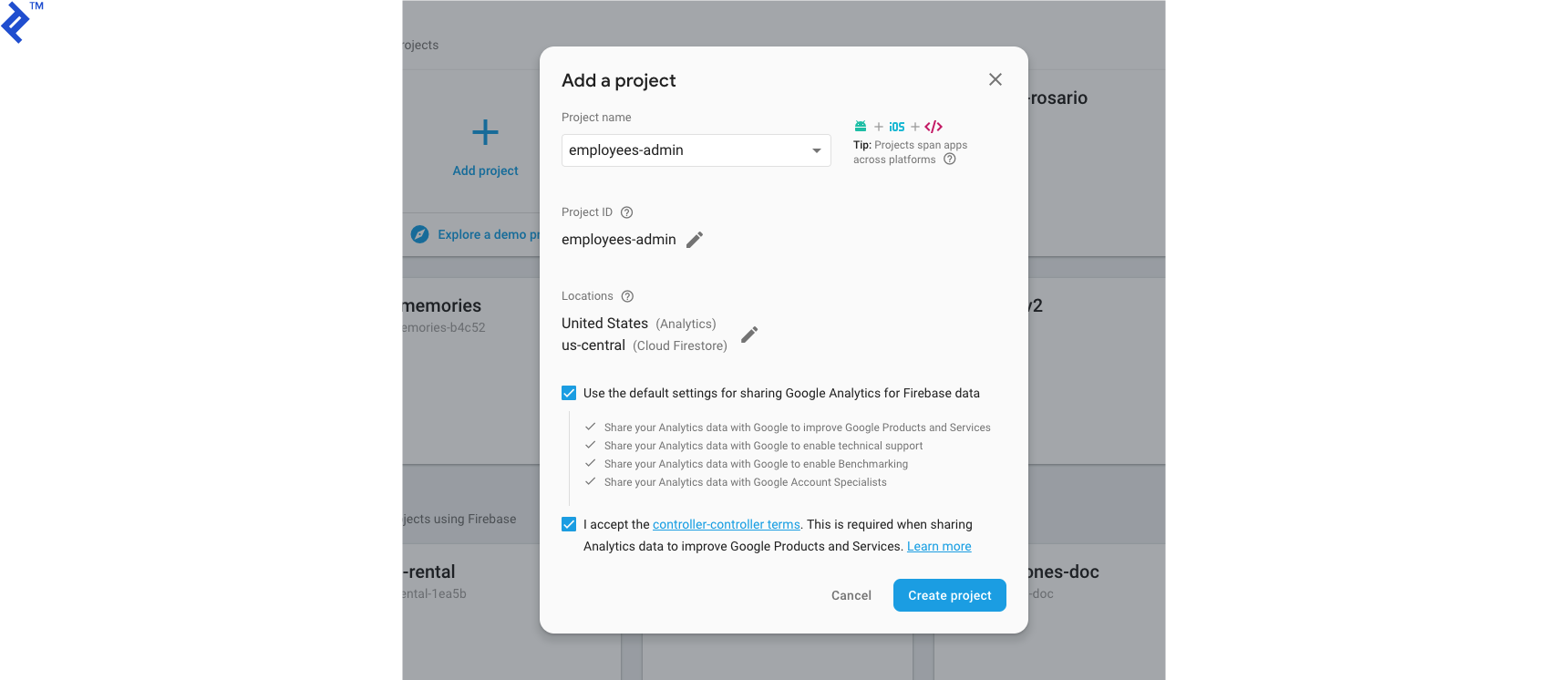The image is a screenshot of a web page displaying details for a project configuration. 

In the upper left-hand corner, there is an option labeled "Add a project". Below this, the "Project name" section is filled with the name "employees-admin". Adjacent to the project name entry, a tooltip reads: "Project span apps across platforms".

Further down, the "Project ID" is also listed as "employees-admin". The "Location" is set to "United States", and "Analytics" points to "US-Central Cloud Firestore".

Beneath these entries, there's an option to utilize the default sharing settings for Google Analytics for Firebase data, which is turned on. A small print below explains several sharing options with Google:

- Share your Analytics data with Google to improve Google products and services.
- Share your Analytics data with Google to enable technical support.
- Share your Analytics data with Google to enable benchmarking.
- Share your Analytics data with Google account specialists.

At the bottom, there is a requirement to accept the controller-controller terms when sharing Analytics data to improve Google products and services.